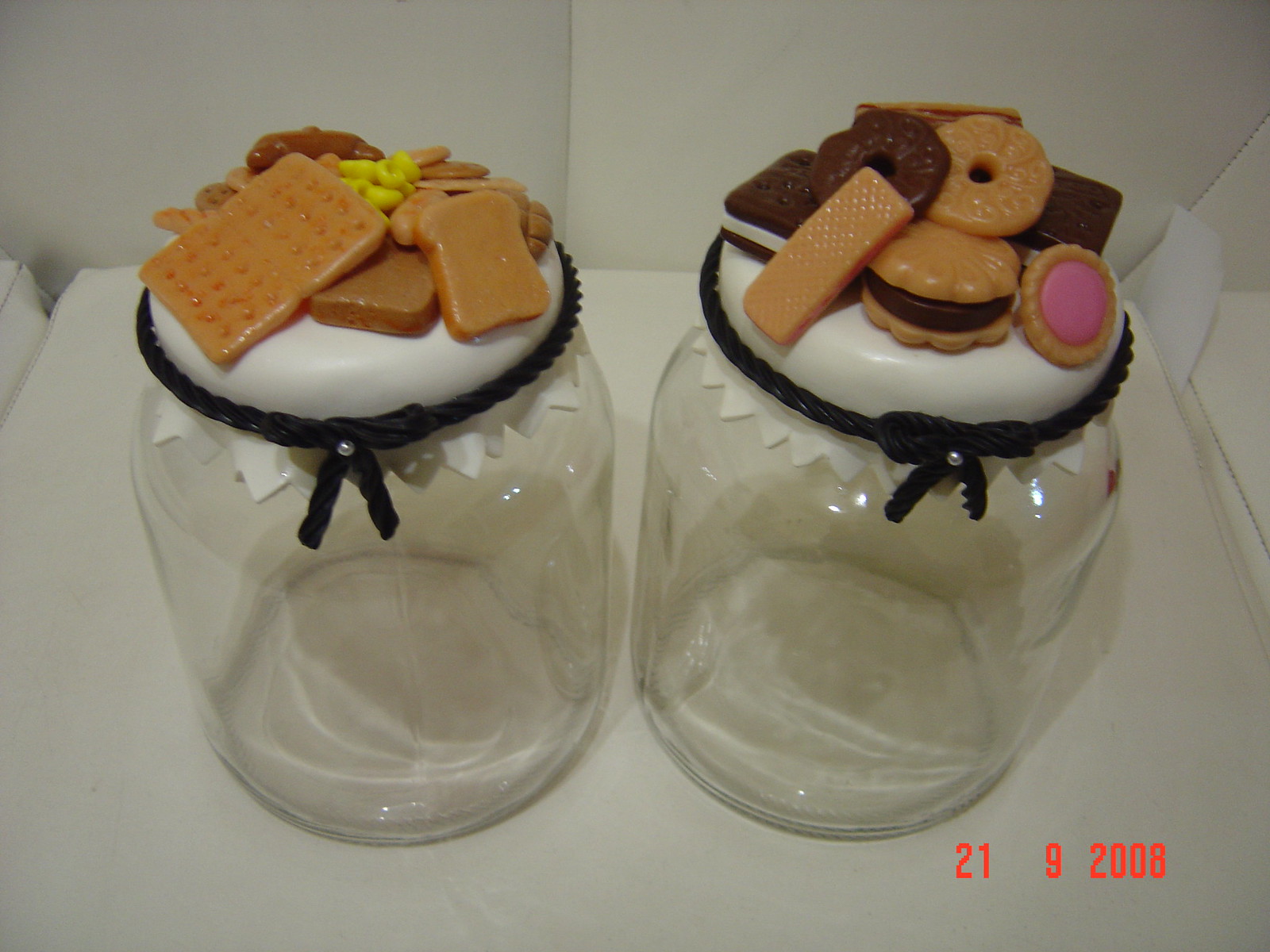The photograph, timestamped 21-9-2008 in red text, captures an indoor setting featuring two empty, evenly cylindrical glass jars placed horizontally on a white surface, which appears to be a couch cushion. These jars, identical in their plain glass design, stand out due to their ornate lids. Each lid is encircled by a black ribbon tied into a bow, complete with a pearl in the center. Atop these lids lie intricate plastic decorations mimicking an array of baked goods. The left jar's lid showcases two large graham crackers, a piece of toast, and an additional yellow feature in its center. The right jar's lid displays a single biscuit alongside a more complex arrangement, including an ice cream sandwich-like treat, two circular biscuits on top of a sandwich with brown filling, and a beige disc with pink filling. The background reveals another cushion, adding to the cozy, domestic atmosphere of the image.